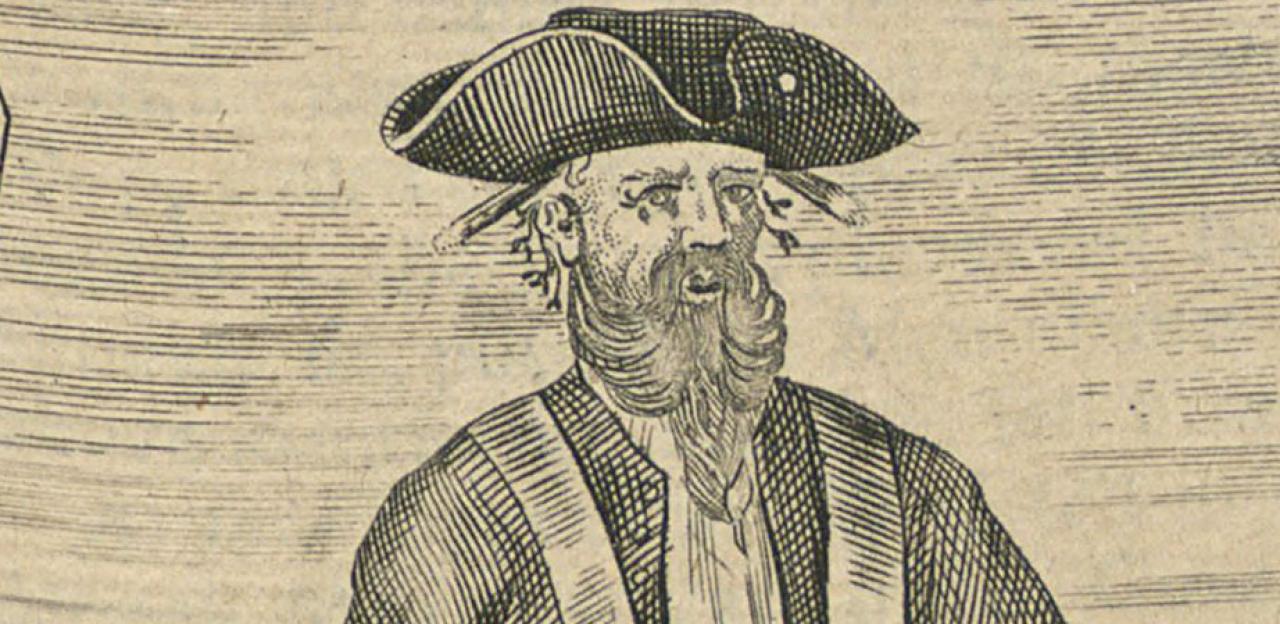This image is an intricately detailed pen or pencil drawing rendered in black fine lines on a background that is aged, appearing beige or tan in color. The background of the image features thin, faded lines which may represent stylized clouds or patterns, giving it an old-timey feel reminiscent of antique newspapers. 

At the center of this artwork is a man whose head and shoulders dominate the composition. He wears a commanding hat, similar in style to those worn by pirates or naval officers, which narrows to a tip at the front and broadens at the sides. Emerging from the underside of this hat are peculiar twig- or branch-like elements, adding an enigmatic touch to his appearance.

The man has a prominent nose and his mouth is slightly open. His eyes, with a possible scar-like marking near his left eye, lend character to his composed yet rugged expression. His facial hair is striking—a long, wavy beard that tapers to a fluffy point and a mustache with curled edges. 

He dons a coat marked by striped patterns, hinting at a military or naval influence, though the garment remains partially obscure. His facial features and attire, combined with the mysterious elements and fine linework, create a rich visual narrative within the confines of the monochromatic, aged paper.